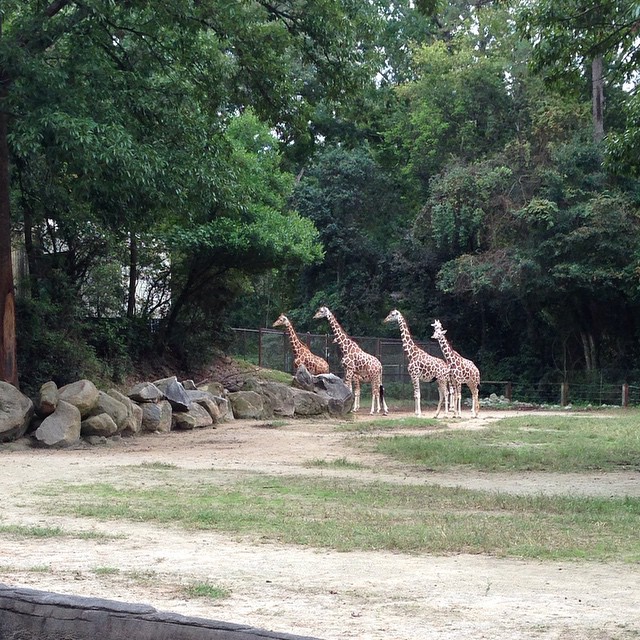This outdoor photograph, likely taken at a zoo or animal sanctuary, features five giraffes standing close together, with their attention drawn towards the left side of the image. The giraffes, most of which are tan with dark chocolate brown spots, are positioned in a dirt and grass-covered enclosure. One giraffe stands out with its deeper chocolate brown hue. Surrounding them, gray, sharp-edged rocks interspersed with green and blue accents line the ground, leading up to a dense array of dark and light green trees that edge the left side and continue to the right. The enclosure is partly bordered by a concrete stone wall visible in the lower left-hand corner, contrasting with the natural setting. The ground, predominantly dirt with sandy patches, displays worn paths presumably created by the wandering giraffes. A piece of wood serves as a barrier in the foreground. In the distance, fences can be seen, reinforcing the zoo-like environment, and it appears to be a sunny day with a clear blue sky.